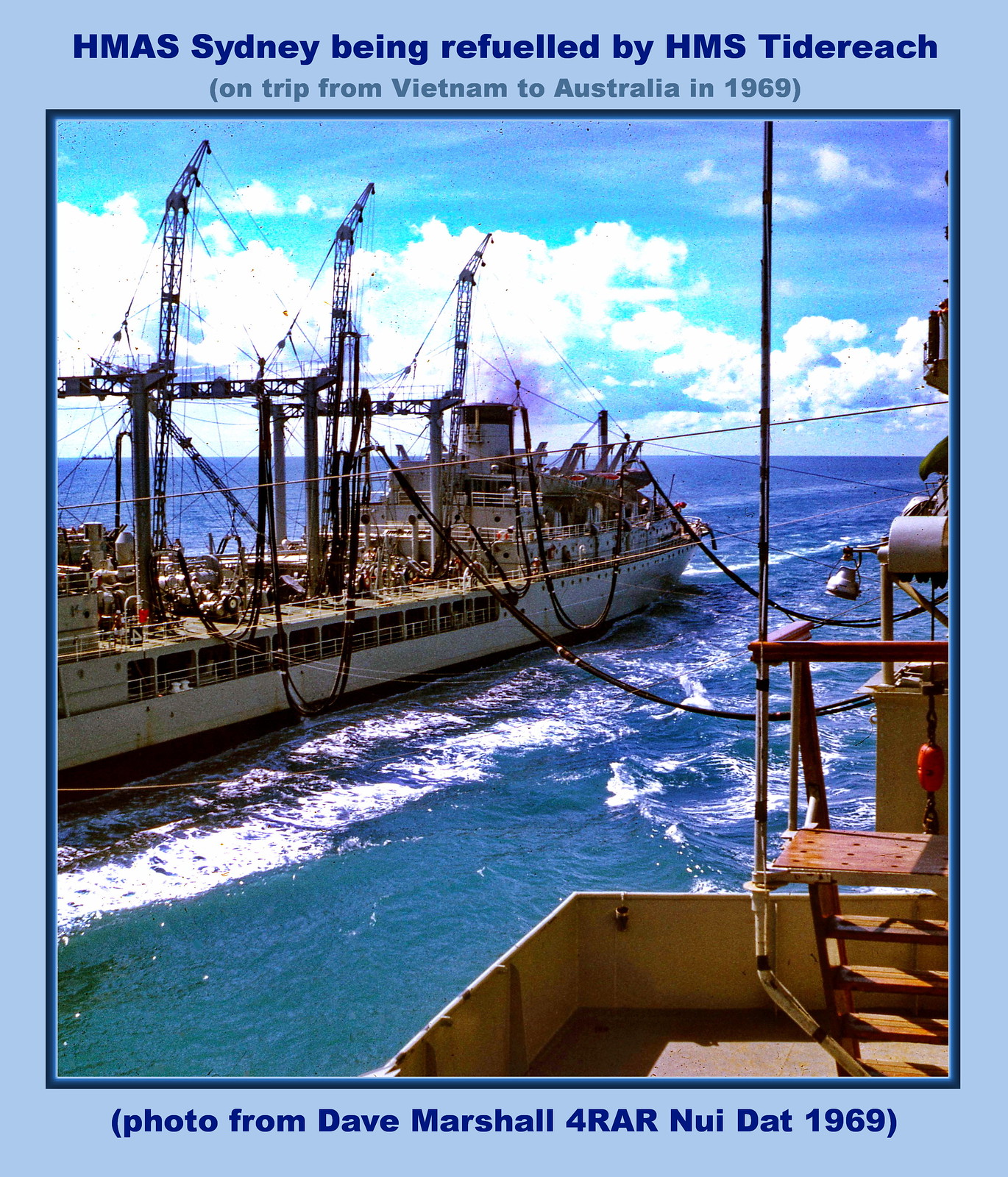This photograph, framed with a light blue border, resembles a vintage postcard. Within the border, the top features dark blue text reading "HMAS Sydney being refueled by HMS Tide Reach," with a subscript in gray text stating, "on trip from Vietnam to Australia in 1969." At the bottom, dark blue text provides, "Photo from Dave Marshall for RAR Nui Dat 1969." The image centers on two ships at sea, with the primary vessel, a weathered white ship showing signs of rust and dirt, situated on the left. This ship, equipped with tall structures that resemble cranes, appears to be receiving fuel from the second ship, partially visible on the right. The scene is bustling with large ropes connecting the ships, machinery, and numerous personnel. The backdrop is a partly cloudy daytime sky.